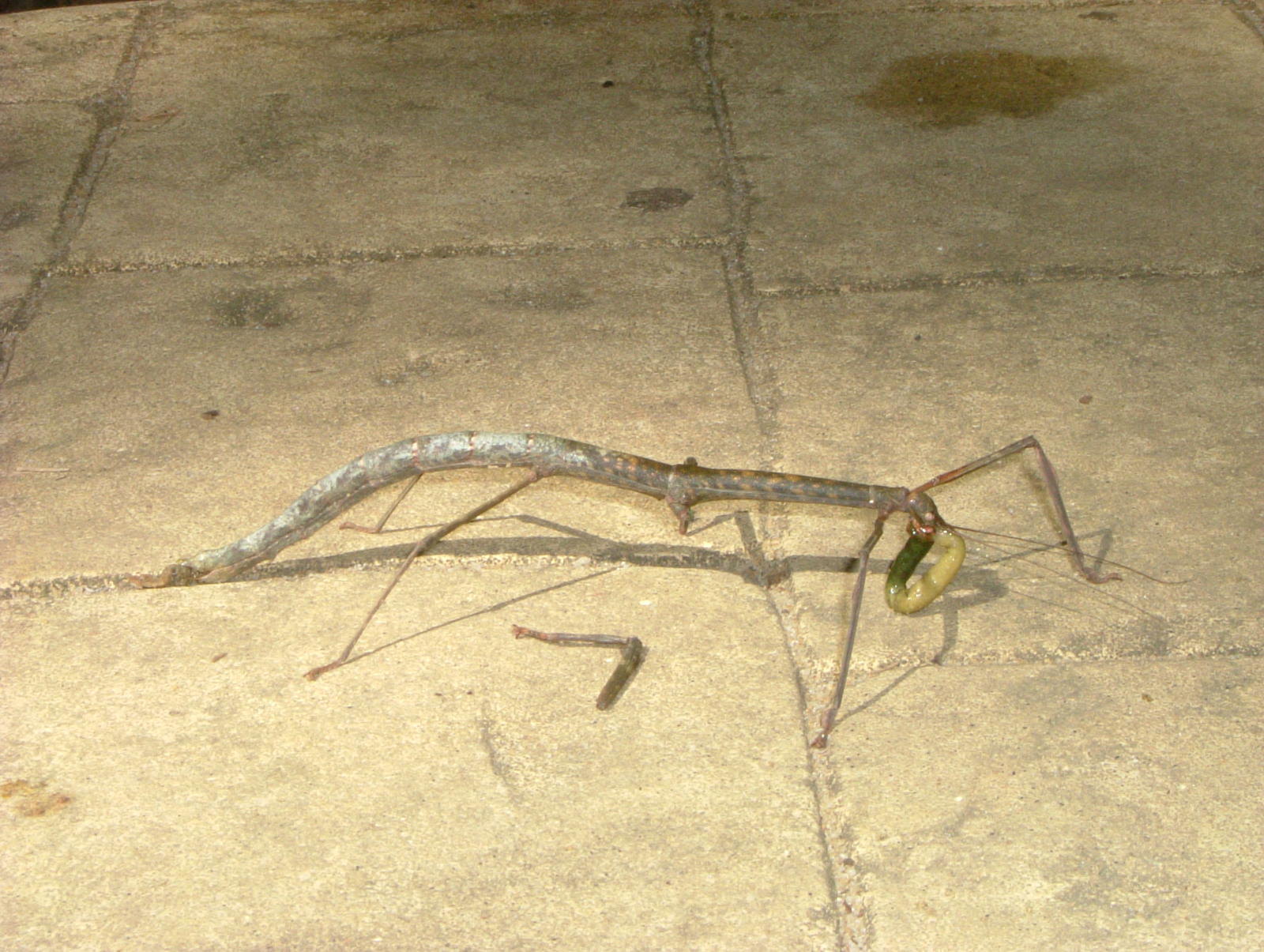A stick bug, resembling a twig with thin branches, traverses a path of desaturated yellow-brown stone tiles. The insect's slender legs and antennae, extending delicately from its body, blend seamlessly with its earthy tones, much like the branch of a tree. A green appendage, with hues transitioning from dark to light green, curls around, possibly near its face. The head of the insect, oval-shaped and partially cream and green, contrasts subtly against the stone, suggesting it might be nibbling on another insect. The scene is illuminated by a soft spotlight, enhancing the insect's shadow on the uneven tiling. A distinct yellow stain is visible in the upper right-hand corner of the walkway.